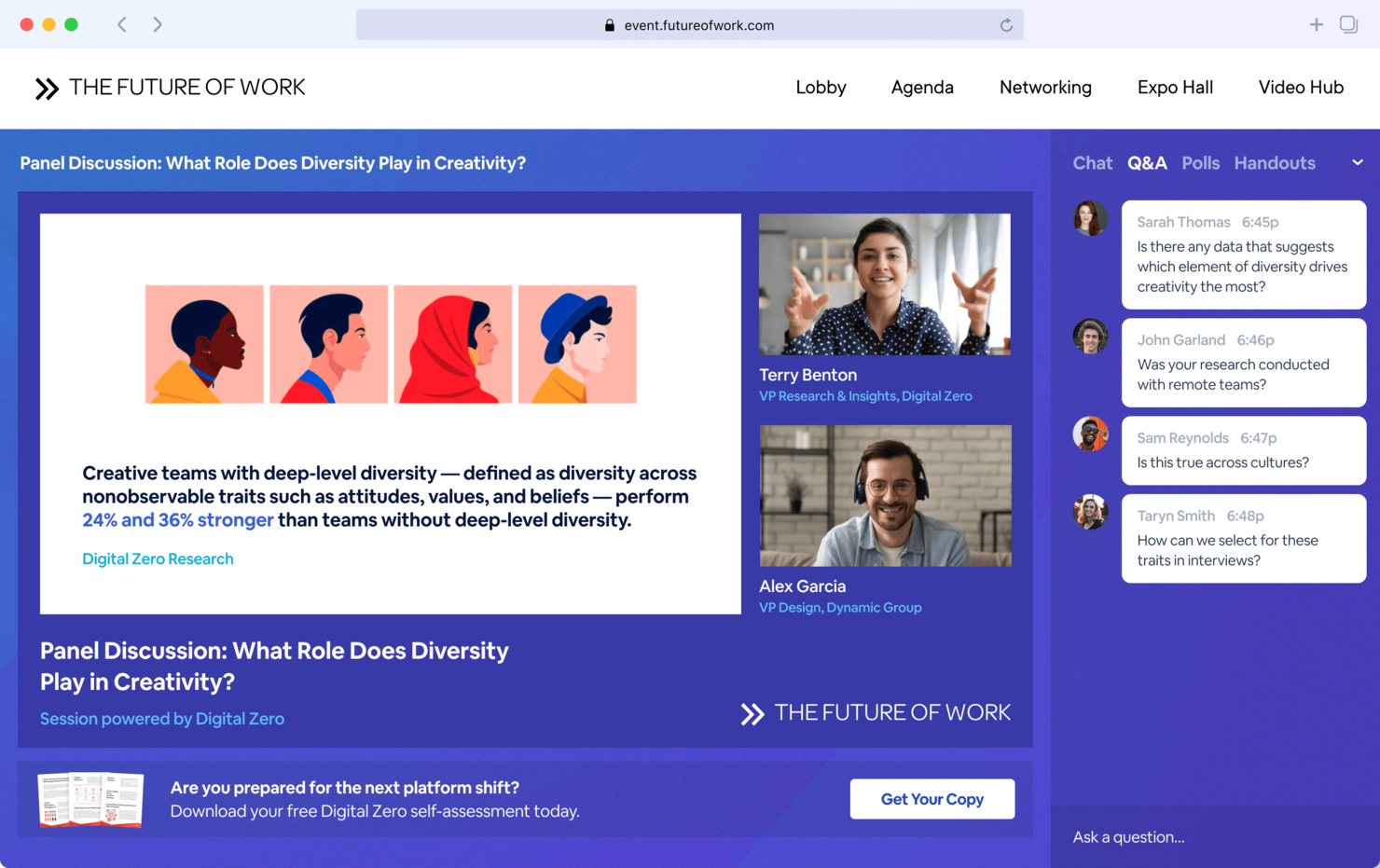Caption: 

A detailed screenshot from the webpage event.futureofwork.com showcases a virtual panel discussion titled "What Role Does Diversity Play in Creativity?". The interface prominently features the event’s navigation menu with tabs labeled 'Lobby,' 'Agenda,' 'Networking,' 'Expo Hall,' and 'Video Hub.'

Centrally, an artistic depiction of four diverse individuals—representing various genders and ethnicities—illustrates the topic’s focus on diversity. Text within the image highlights key research findings, stating, "Creative teams with deep-level diversity, defined as diversity across non-observable traits such as attitudes, values, and beliefs, perform 24% and 36% stronger than teams without deep-level diversity." This insight is attributed to Digital Zero Research.

The session is sponsored by Digital Zero, encouraging viewers to download a "free Digital Zero self-assessment" to prepare for future work shifts. The event also showcases key speakers including Terry Benton, VP of Research and Insights at Digital Zero, depicted as a young woman smiling with hands raised, and Alex Garcia, VP of Design at Dynamic Group, portrayed wearing headphones, glasses, and sporting facial hair.

To the right of the image is an interactive panel displaying chat functionalities with tabs for 'Chat,' 'Q&A' (which is selected), 'Polls,' and 'Handouts.' Several question inputs by participants are visible, such as Sarah Thomas inquiring about data on elements of diversity driving creativity, John Garwin questioning the context of the research with remote teams, Sam Rimmel asking about cross-cultural applicability, and Taryn Smith seeking advice on how to select for these traits in interviews, with timestamps for each entry provided. The panel also includes an "Ask a Question" feature, allowing attendees to actively engage with the discussion.